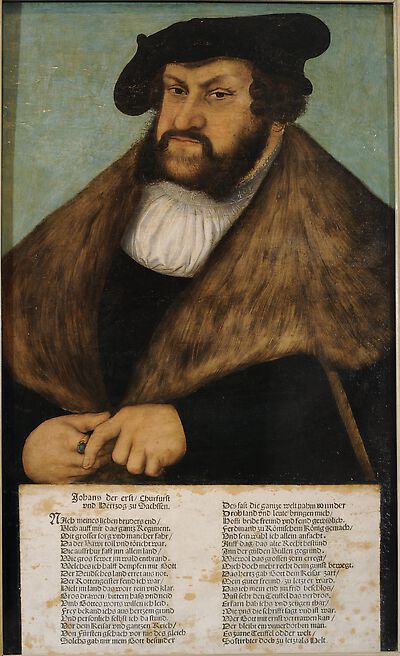This Renaissance-era painting features a portly and stout man sitting and posing with an air of composed dignity. He has dark, curly hair that reaches mid-ear, complemented by a beard and prominent mutton chops framing his round face. His attire includes a black French-style beret and a luxurious heavy overcoat with a large, dark brown fur collar. Underneath, he wears a white, ruffled high-necked shirt that adds to his dignified appearance. 

At the bottom of the painting, there is a graphic display of cursive text, likely written in a Renaissance-era language that is not English. The background of the painting is a serene greenish-blue, providing a calming contrast to his striking presence.

The man is clasping his hands in front of him, with a notable gold ring featuring a green stone on the index finger of his left hand. His facial features include a long nose, subtly squinting eyes, and an underbite. While he is not smiling, his expression is neutral, exuding neither sternness nor cheerfulness, but perhaps a reserved wisdom. This detailed and meticulously composed portrait captures the essence of a prominent figure from the Renaissance period.